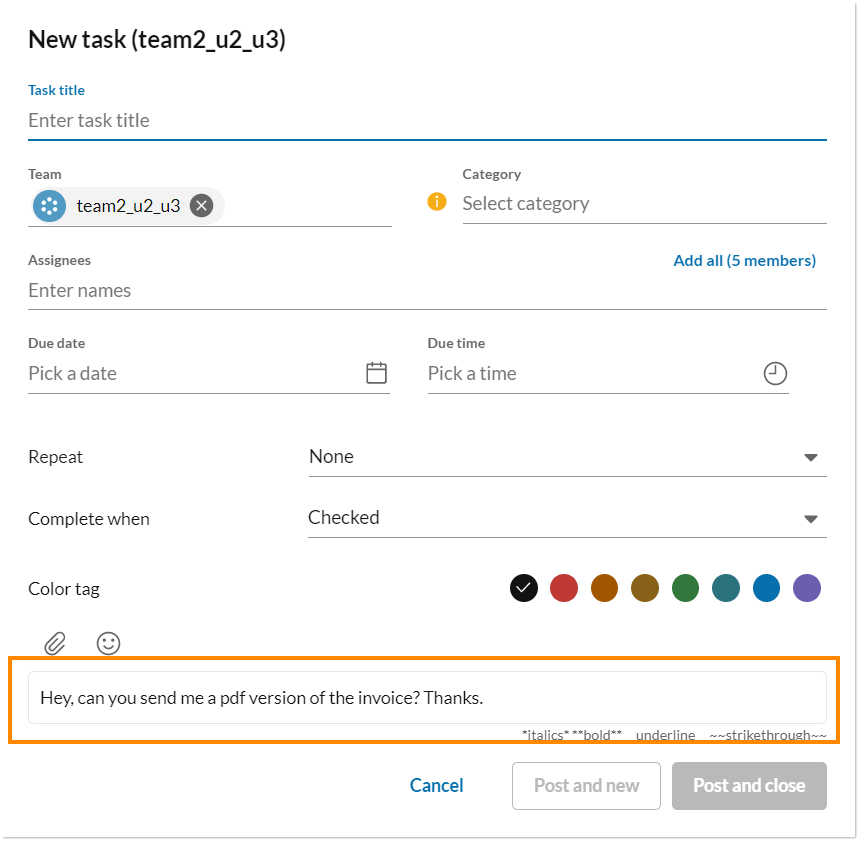**Caption:**

A detailed screenshot of a task management interface.

In the upper left-hand corner, bold black text reads *"New Task (Team2_U2_U3)."* Below, in blue text, is the label *"Task Title,"* followed by *"Enter Task Title"* in yellow. A long blue line stretches horizontally across the screen.

Underneath the line, the word *"Team"* appears, and below it is a horizontally-oriented gray oval area. This oval contains a blue, round, wheel-like icon on its left. In the center of the oval, the text reads *"Team2_U2_U3"* with an 'X' inside a black circle to the right.

To the right of the Team section, the label *"Category"* is displayed with the text *"Select Category"* and a yellow information icon ('i'). Below, several fields are listed for assigning the task:
- *"Assignees:"* Enter Names, Add All 5 Members
- *"Pick a Date:"* Due Date, Pick a Date
- *"Due Time:"* Pick a Time (with a clock icon next to it)
- *"Repeat:"* None
- *"Complete When Checked"*
- *"Color Tag:"* (followed by a horizontal line of different colored circles; a black circle has a check mark in its center)

At the bottom, a message reads: *"Hey, can you send me a PDF version of the invoice? Thanks."*